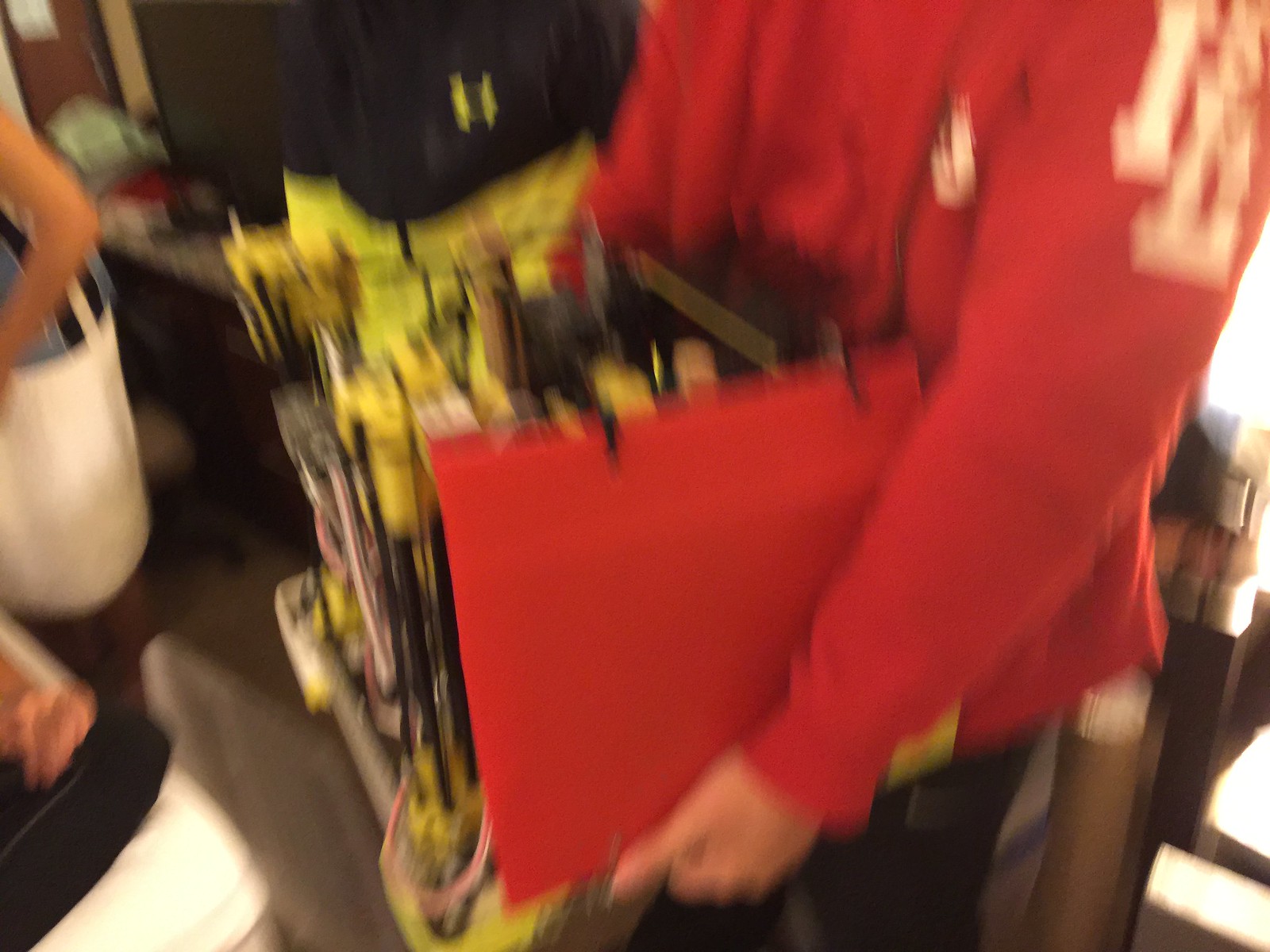The photograph, notably out of focus and blurry, is centered on a figure likely to be a Caucasian male. He is clad in a red hoodie adorned with unreadable white lettering on the sleeve and chest. The photo captures his torso down to about his thighs, and he is holding a red container or box filled with indistinct black and yellow items. The image suggests movement at the time it was taken, contributing to the overall blur, and is wider than it is tall. Additional details include glimpses of other people: a visible elbow of a woman in the far left and perhaps a foot in the lower left. The background contains another partial view of an individual, identifiable by a white skirt and a blue top with a navy stripe.